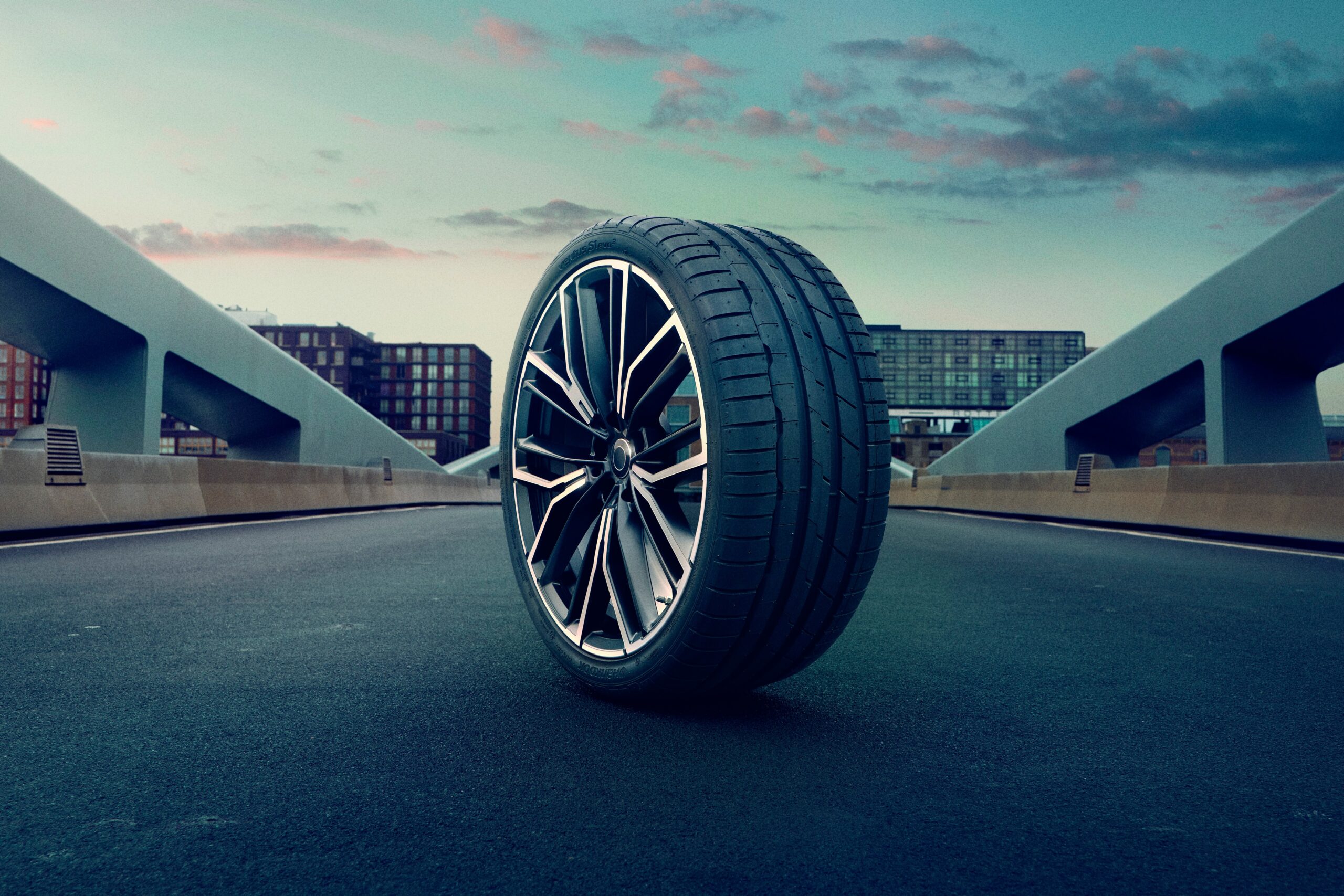In a striking image resembling artwork, a lone car tire stands upright on a dark black cement road, flanked by short dark gray concrete barriers. Behind these barriers are taller, light grayish-blue walls that slope upward, reminiscent of bridge inclines. The scene appears to be at the cusp of sunset, with a sky transitioning from light on the left to a deeper blue on the right, interspersed with streaks of purple, dark pink, and gray clouds. In the distance, dark gray multi-storied buildings rise prominently. The tire is black rubber with chrome spokes radiating from the center, forming five distinct double lines that split midway towards the rim. The setting exudes an air of urban solitude and surrealism, as if the tire has embarked on a solitary journey amidst the concrete and steel surroundings.